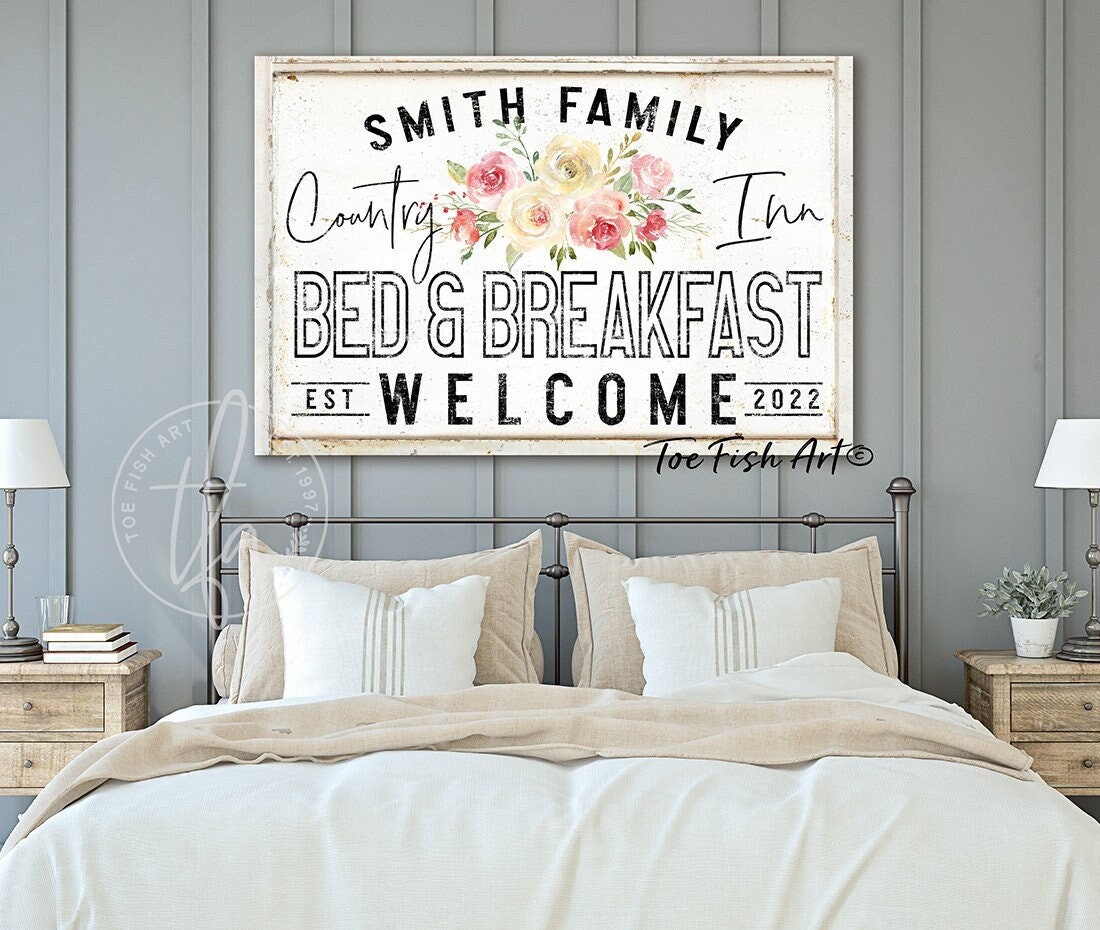In this square, daylight photograph of a meticulously arranged bedroom, we see a warm and inviting ambiance. The focal point is a stylishly adorned bed with a brushed silver metal headboard, positioned against a vertical gray paneled wall. The bedding ensemble includes a white blanket and beige-colored covers, flanked by two tan pillows and two white and tan-striped throw pillows, creating a cozy and harmonious look.

Above the bed, a large, horizontal rectangular wooden sign, weathered white with natural brown accents, prominently features black, all-caps text reading, "Smith Family," followed by "Country Inn" below it. Nestled between "Country" and "Inn" is a vivid arrangement of pink, white, and yellow flowers with green leaves. Further down, the sign continues with "Bed and Breakfast" in black block letters. At the bottom, it reads "EST 2022," framed by lines above and below, with a bold "Welcome" in the center. The sign also bears the digital watermark "Tow Fish Art ©" and an additional logo indicating "Tow Fish Art Established 1997," subtly blended into the image.

Flanking the bed are two natural wood nightstands. The left nightstand hosts a few books, a clear water glass, and a lamp, while the right one features a potted plant and another lamp, complementing the room's cozy and inviting feel. The carefully curated details and decor elements make this bedroom a serene and welcoming retreat.